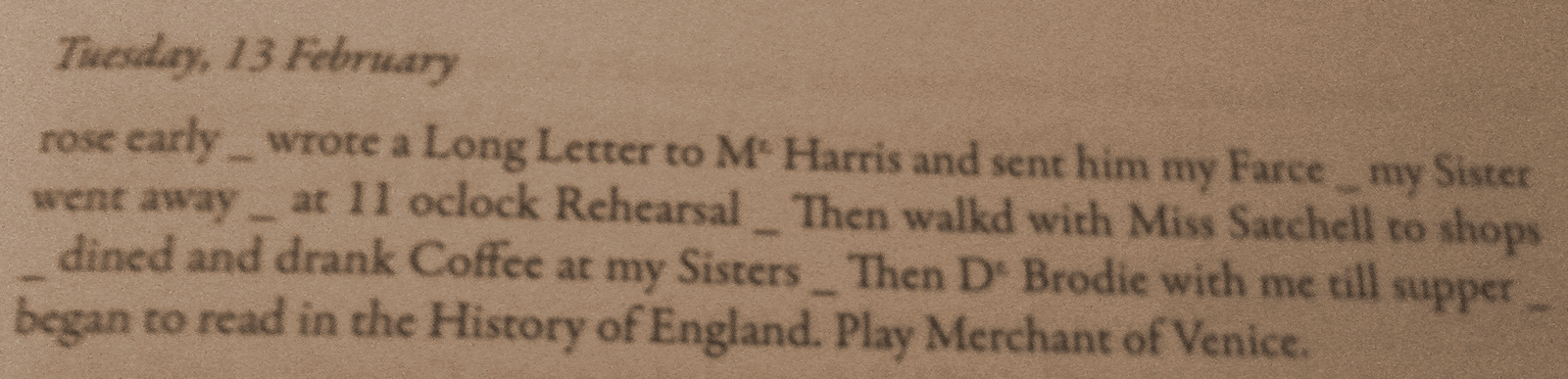In this image, there are no actual objects present. Instead, it appears to be a snippet from an old newspaper or book, taking up nearly the entire frame. The background is a tannish or brown color, and the text is typed in black. The date "Tuesday, 13 February" is at the top left, written in italics, suggesting a potential diary entry or dated note. The text beneath the date is fragmented and reads: "Rose early wrote a long letter to Harris and sent him my farce. My sister went away at 11 o'clock. Rehearsal, then walked with Miss Satchel to shops, dined, and drank coffee at my sister's. Then de Brody with me till supper. Began to read in the history of England. Play Merchant of Venice." The overall style is reminiscent of an old, handwritten or typed document, capturing a daily log or personal note.